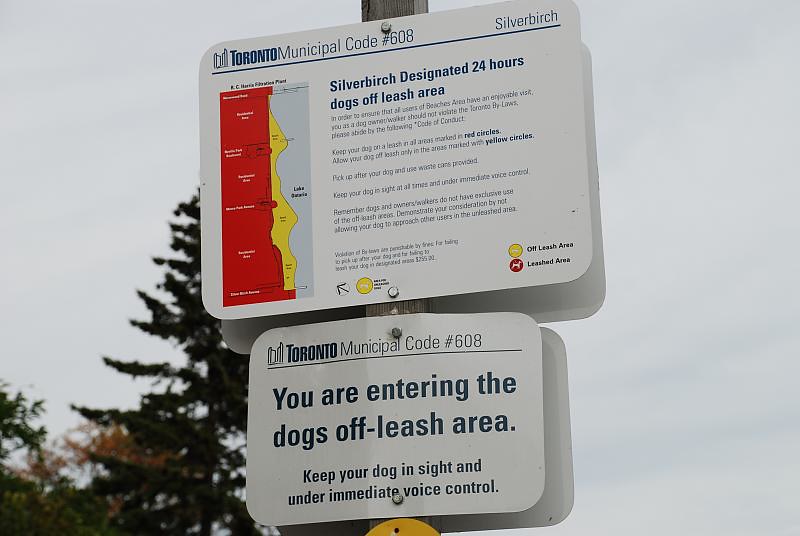The image captures two rectangular metal signs attached to a wooden pole, likely located in Canada, as suggested by the mention of "Toronto Municipal Code 608." The top sign, slightly larger with a white background and blue text, reads: "Toronto Municipal Code 608. Silver Birch. Silver Birch designated 24-hour dogs off-leash area." This sign includes a map with red and yellow wavy sections denoting areas where dogs must be leashed (red) and where they can be off-leash (yellow). Additionally, there's a yellow circle indicating an off-leash area and a red circle for leashed areas. The bottom sign echoes the code number and provides further instructions: "You are entering the dogs off-leash area. Keep your dog in sight and under immediate voice control." The background reveals a cloudy sky and evergreen trees to the left, suggesting a bright but overcast day.